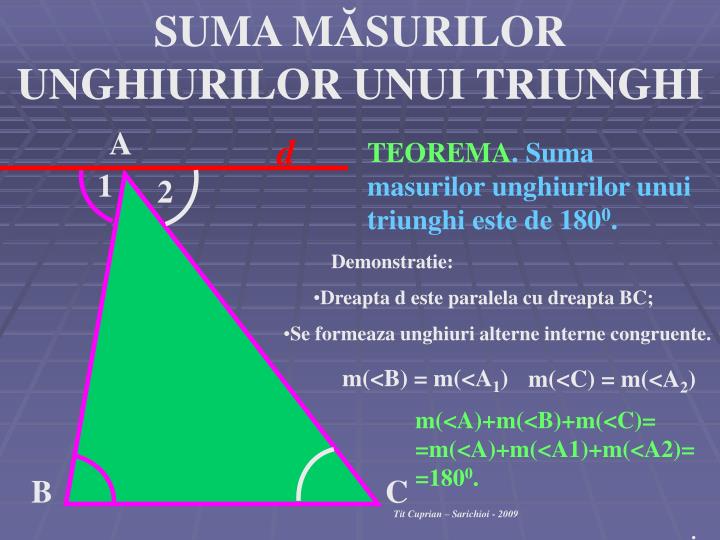The slide appears to be part of a PowerPoint presentation with a background composed of blue and purplish-blue squares. At the top, there is a title in white, all caps letters, centered and reading: "SUMMASURILOR UNGHIURILOR UNUITRIUNGHI." Below the title, on the left side of the slide, there is a green triangle with a purple outline. The triangle's top angle is labeled 'A' and flanked by the numbers '1' and '2'. A red horizontal line intersects the top of the triangle and is labeled 'D' in red. Each point of the triangle is marked with letters: the top is 'A', the bottom left is 'B' (in purple), and the bottom right is 'C' (in white). On the right side of the slide, there is green text stating "TEOREMA," followed by more blue text and smaller white text with bullet points and equations at the bottom. The content and text on the slide are in a foreign language, distinctively different from English.